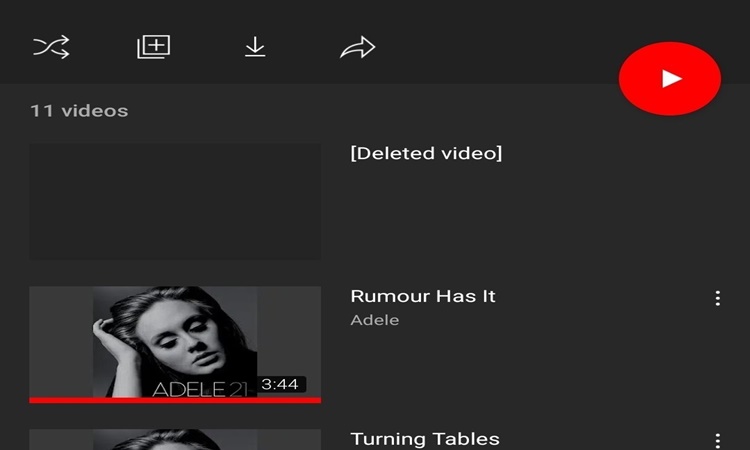This is a screenshot of a YouTube section, possibly related to Adele, though it's unclear if it's her official page given the limited content. The top of the page features several symbols for sharing, adding videos, uploading, and downloading, followed by the text "11 videos." To the right, the YouTube logo appears. 

Two videos are partially visible. The first is titled "Rumor Has It" by Adele, with a duration of 3 minutes and 44 seconds. It displays the black and white album cover and indicates it has already been played, highlighted by a red progress bar. The second video is named "Turning Tables," but it lacks any visual elements, suggesting it might be a deleted or unavailable video.

The rest of the page below this point appears empty, aside from showing the total count of 11 videos, though only these two—one partially titled and one "deleted video"—are visible in this snippet. In the lower part, there's a brief explanatory note indicating that one video had content, while another was deleted.